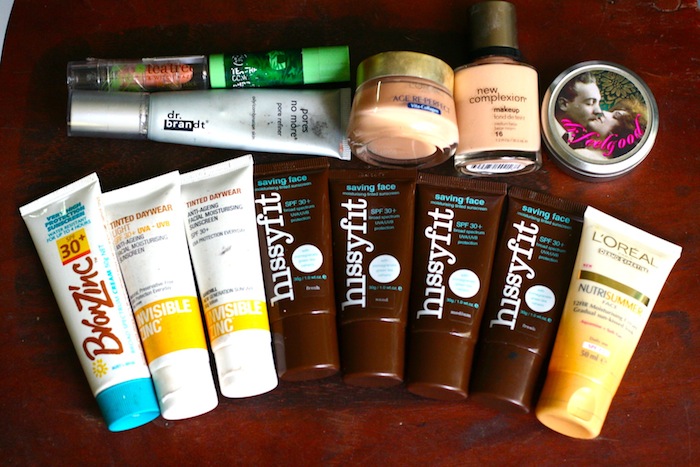The photograph showcases a variety of makeup and skincare products arranged in a neat display. At the bottom, there is an arc of eight tubes, which appear to be different types of suntan lotion and skincare items. The first tube, labeled "Bronze Zinc," is likely a suntan lotion with an SPF of 30+. Next to it are two identical tubes of "Invisible Zinc," which are white with a gold band, hinting that they might also be sunscreen products.

Following these are four brown tubes labeled "Hissy Fit" in white lettering, with "Saving Face" highlighted in blue at the top, also marked with SPF 30+. These too seem to be suntan lotions. The final tube in this row is a "L'Oreal Nutra" product, though the exact type isn’t clear, it might be another skincare item.

Above these on the left, there is a branded tube labeled "Dr. Brandt." Above this tube are two smaller tubes that appear to be lip glosses or chapsticks; one has a pinkish hue, while the other comes in a green container. 

Adjacent to these, there is a small glass tub with a gold-rimmed cap, though its contents are uncertain. The next item in line is a small bottle labeled "New Complexion Makeup," indicating it’s a type of foundation or facial makeup. 

Finishing off the display is a circular container featuring an illustration of a man and woman kissing, the label of which remains unreadable. The diverse collection highlights various products focused on skincare and beauty.